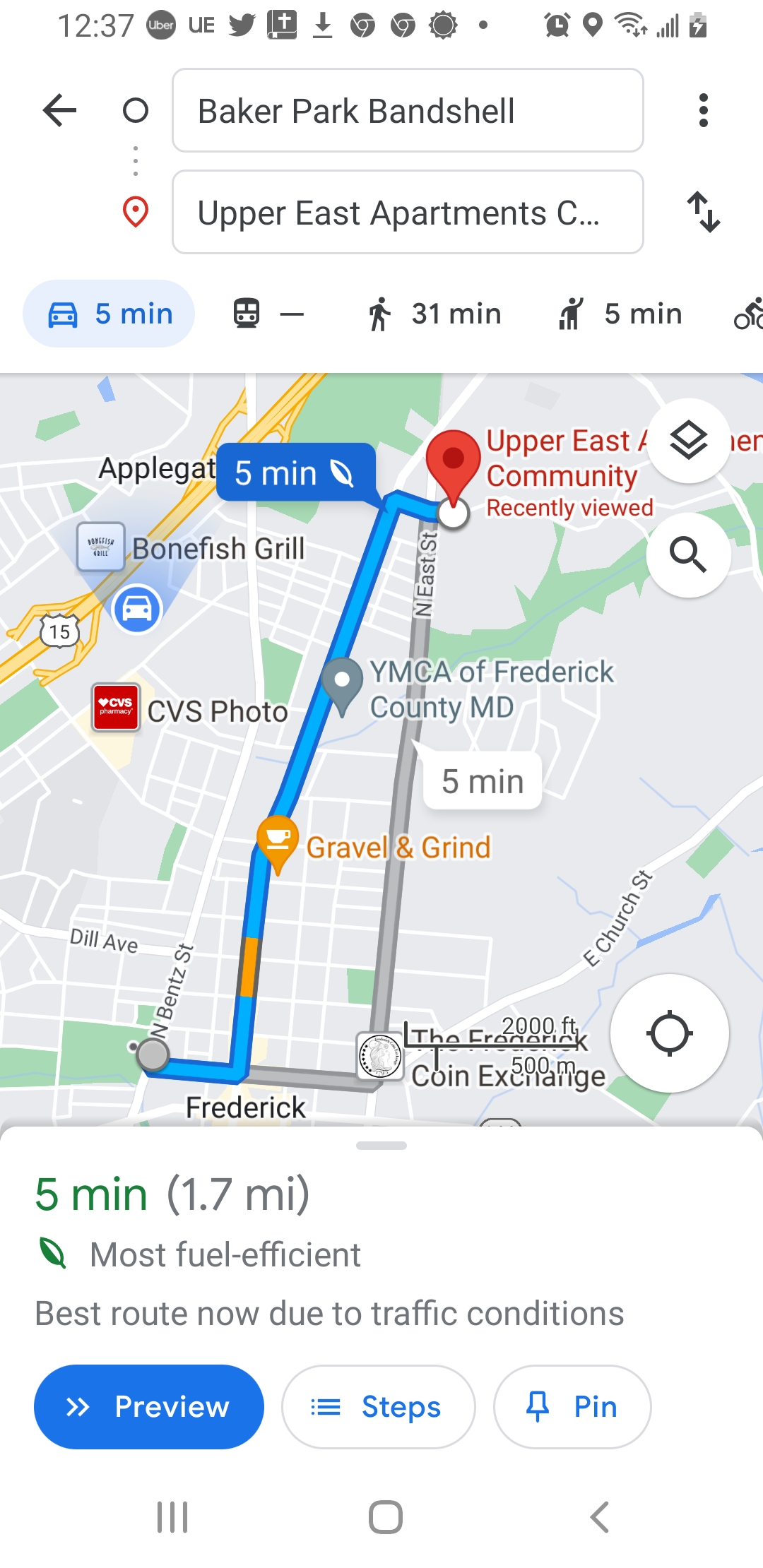This is a screenshot from the Google Maps app displayed on a mobile phone, presenting driving directions from Baker Park Bandshell to Upper East Apartments in Frederick County, Maryland. The main driving route is highlighted in blue and spans a distance of 1.7 miles, estimated to take five minutes. An alternate route is depicted in gray. Key landmarks labeled on the map include a CVS Pharmacy, Bonefish Grill, and the YMCA of Frederick County, Maryland. The phrase "most fuel efficient" is also noted at the bottom of the screen.